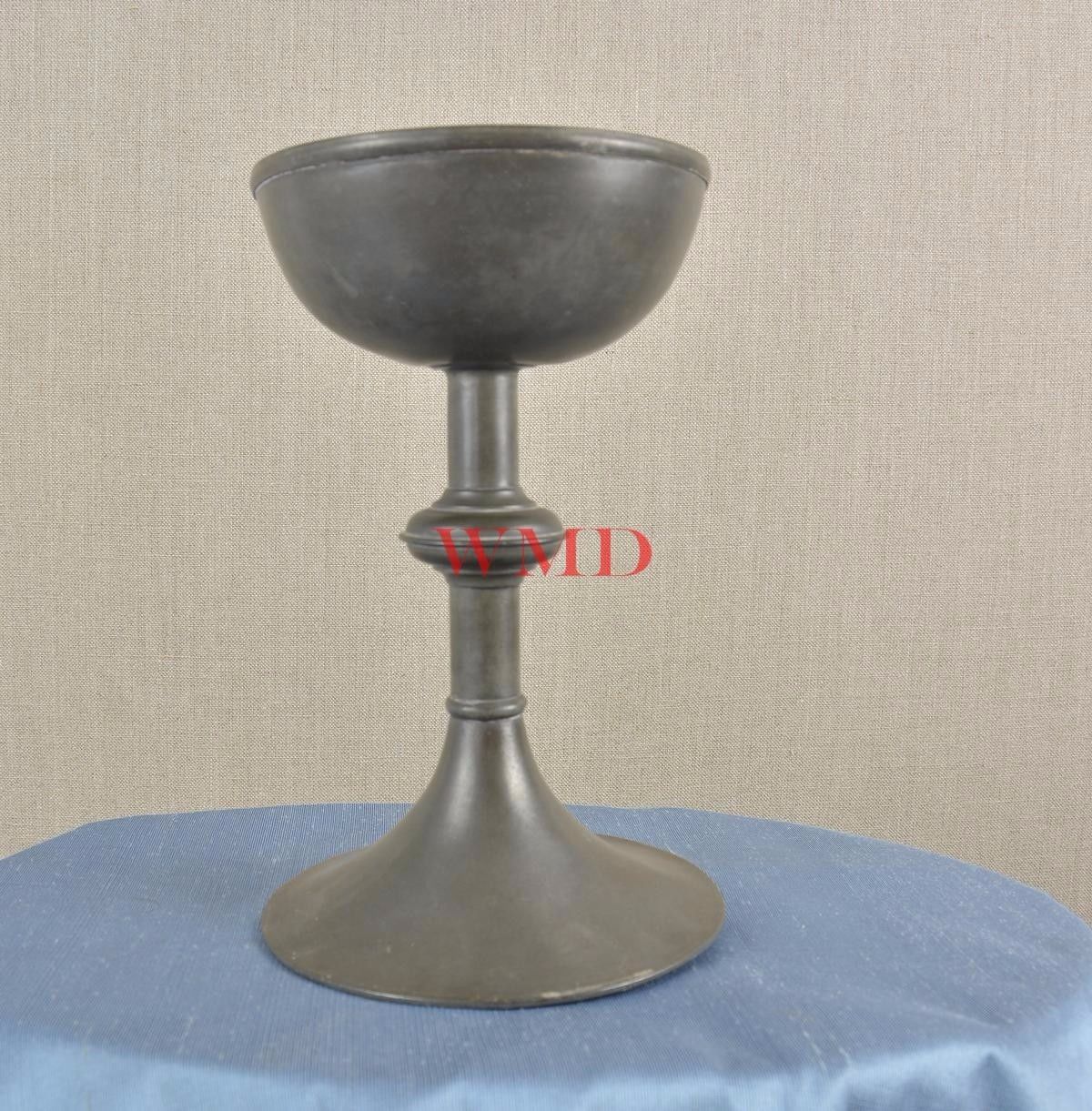This photograph features a minimalist scene with a light beige wall in the background, covered in textured, fabric-like wallpaper. Centrally positioned is a large, silver metal chalice, reminiscent of a short wine glass, with a flared base and stem. It rests atop a small, round table draped in light blue satin fabric, adding a touch of elegance to the setting. The image is marked with a red watermark in a Times New Roman-like font, displaying the initials "WMD" at the center. The overall composition suggests an air of ritualistic or ceremonial significance.